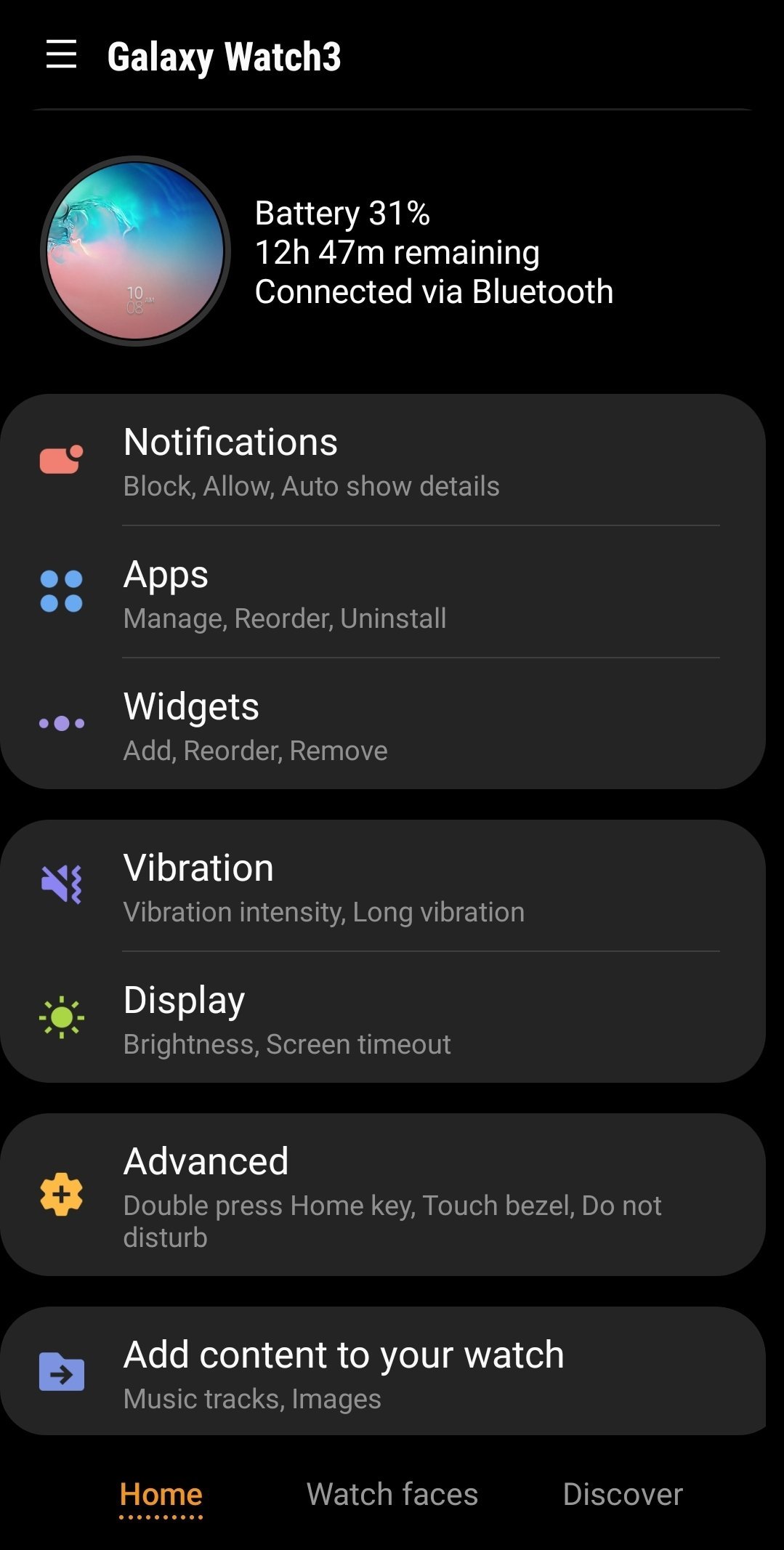This screenshot showcases the settings page for a Galaxy Watch 3, displayed on a smartphone. The background is black, and at the upper left corner, "Settings" is written in white font. Just below, a representation of the watch face appears, characterized by an oval shape with a gradient color scheme—sky blue on the top half and dusty pink on the bottom half. To the right of this, the battery status is shown in white font, indicating "Battery 31%" with "12 hours and 47 minutes remaining," and confirming that the device is connected via Bluetooth.

Further down the page, a series of rectangular sections are displayed in a dark gray color against the black background, each labeled in white font. Listed from top to bottom are: 
- Notifications
- Apps (represented by four blue dots forming a square)
- Widgets
- Vibration (represented by a purple speaker with a line through it)
- Display (represented by a yellow sun-like icon with dots around it)
- Advanced
- Add content to your watch

At the very bottom of the screenshot, there are three options displayed in colored fonts: "Home" in an orange font on the left, "Watch faces" in the center, and "Discover" on the right.